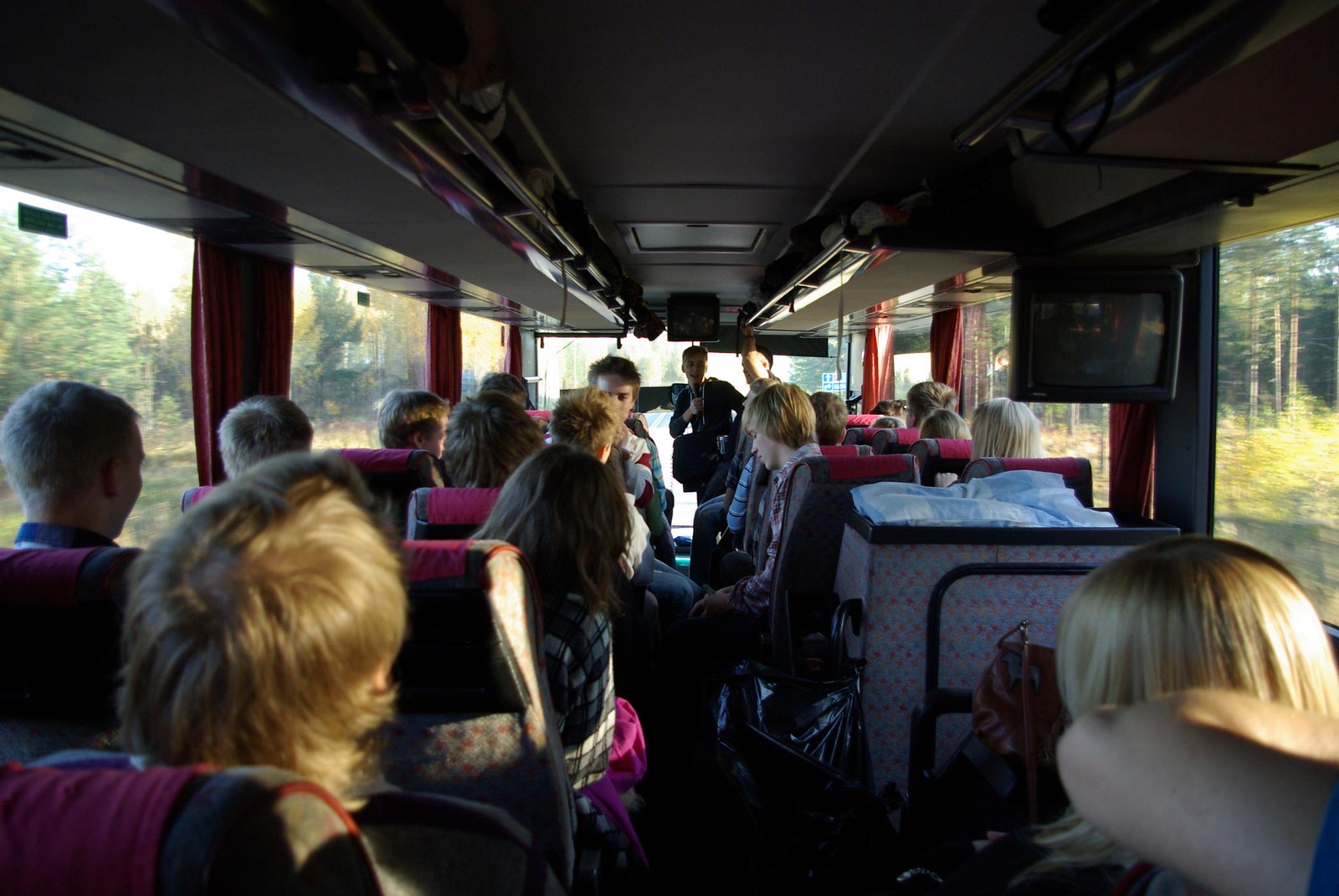The image depicts the interior of a bus, potentially a tour or field trip bus, filled with children, predominantly blonde, with a mix of boys and girls. The bus features rows of seats on both sides, each with a maroon headrest matching the maroon curtains adorning the large, flat-pane windows. Above, luggage racks run along both sides, heavily laden with luggage. On the right side of the ceiling, a TV is mounted. Most children face forward, attentive to a tour guide or teacher at the front, except for a few who appear to be conversing among themselves. One notable figure is a teen in black, possibly addressing the group using a microphone. Outside the large windows, lush green trees are visible, enhancing the scenic backdrop of the journey.